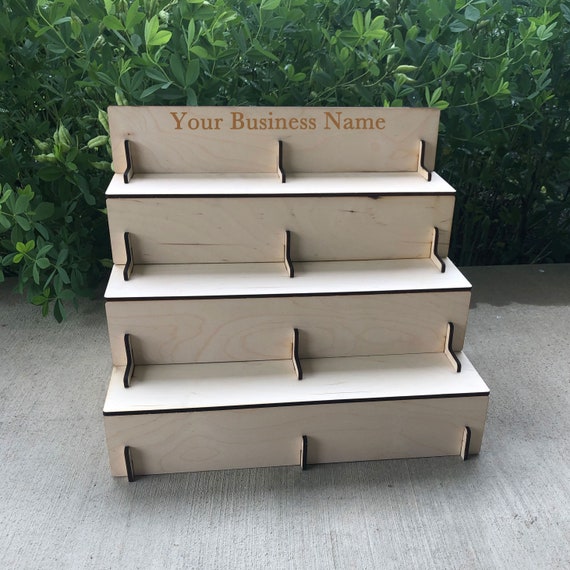The square image, taken outdoors in daylight, features a three-stepped bleacher-style wooden structure positioned centrally on a light gray concrete ground. Crafted from thin, light-colored wood, this homemade shelving unit resembles a set of stairs with standard riser heights. The structure consists of three stairs, with six distinct spaces created by two dividers on each side. At the top, there's a wooden board displaying "your business name" in brown letters, making it customizable. The backdrop is adorned with lush green vegetation, including tall bushes extending over parts of the concrete area, contributing to a vibrant, natural setting.